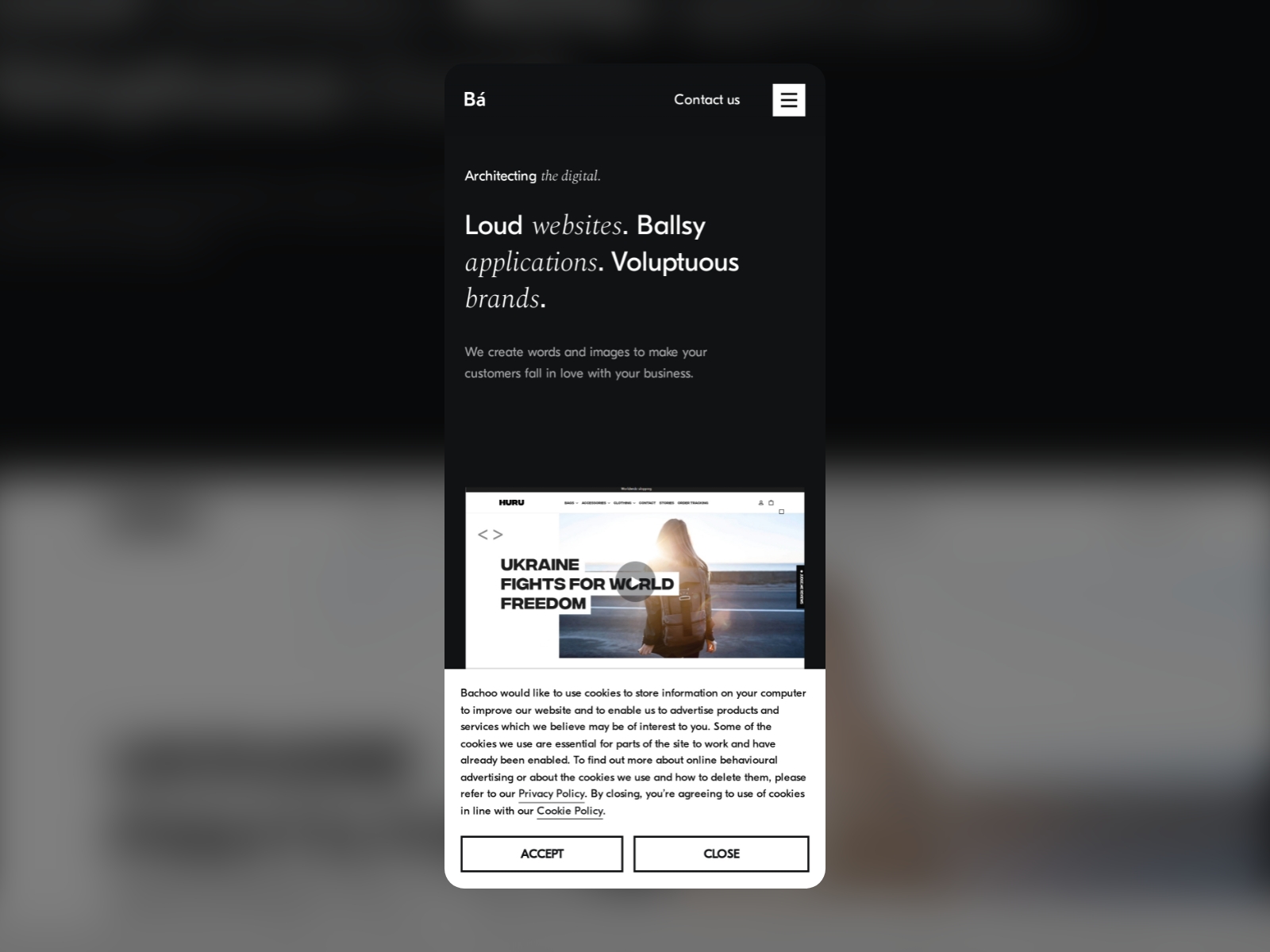The image is a long vertical rectangle with a predominantly black background. In the upper right corner, there is a small white square icon featuring three horizontal black lines next to the text "Contact Us." Further down, the phrase "Architecting the Digital" is prominently displayed, emphasizing the company's focus on building digital solutions. The word "LOUD" is written in bold white text, highlighting their expertise in creating websites. Adjacent to it, "Ballsy" in bold white text stresses their approach to developing applications, followed by "Voluptuous" to describe the brands they craft. 

Beneath these descriptive buzzwords, there is a tagline that reads: "We create words and images to make your customers fall in love with your business." Below this line, there is a clickable video area, indicated by a white arrow in the center. The video preview shows the back of a person with shoulder-length brown hair, dressed in a long-sleeved shirt, standing near a road with a sunset sky in the background.

Further down, there is a poignant message, "Ukraine fights for world freedom," displayed in black text. Beneath this message, a small paragraph in black text, difficult to read due to its size, details additional information. Two underlined options, "Privacy Policy" and "Cookie Policy," are available for further reading. At the very bottom of the image, there are two rectangular buttons with black text; one labeled "Accept" and the other "Close."